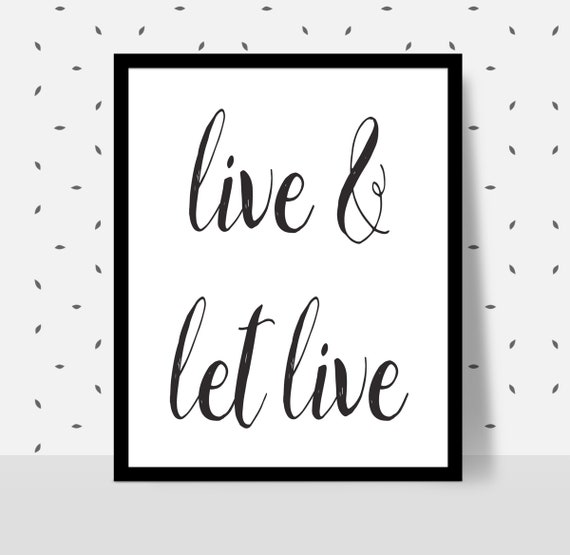The photograph captures a square-shaped image of a digitally created poster hanging on a light gray wall with small black oval-shaped speckles. The bottom section of the wall features a dark gray banner. At the center of the image, a thin black-framed, slightly taller-than-wide rectangular poster displays a white background with elegant, black cursive text split into two lines. The top line reads "Live &" and the bottom line reads "Let Live," with the ampersand symbol used in place of the word "and." The overall aesthetic of the photograph suggests it may be an advertisement for a canvas or a stylized social media post, showcasing the motivational quote "Live & Let Live" against a minimalist and artistically rendered backdrop.